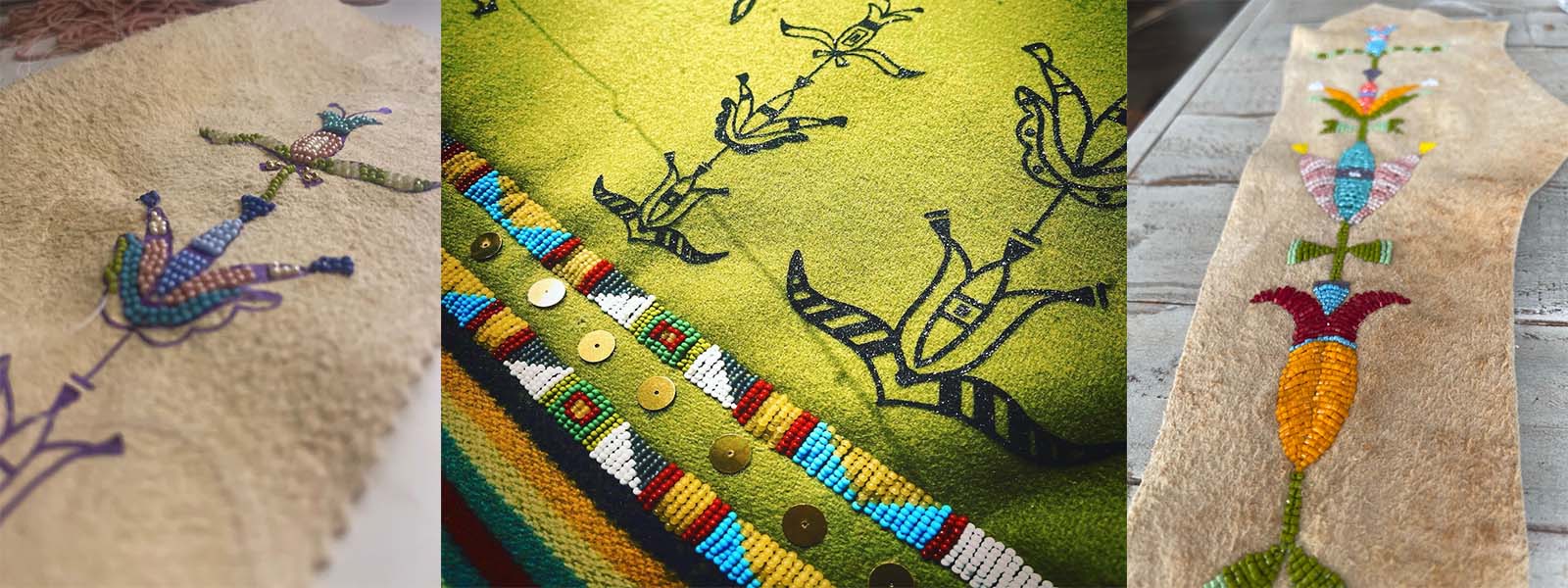This image is a meticulously arranged collage consisting of three rectangular photographs, each about six inches wide and two inches tall. The collage is divided into a left, center, and right section, with the center image slightly wider than the other two. Each photograph showcases intricate beadwork and stitching on fabric that appears to be traditional Native American textile art. 

The left photograph features a light brown or tan fabric, possibly wool or animal skin like deer or cow hide. The fabric has elaborate beadwork in pink, green, and blue hues, as well as purple stitching forming floral patterns. Towards the bottom, additional beading and embroidery extend upward, embellishing the painted designs with beads.

The center photograph highlights a green woolen cloth adorned with painted floral motifs at the top. Black stitching or paint outlines these floral patterns. Diagonal rows of beads, interspersed with buttons, span from the upper left to the lower right, adding a tactile depth to the piece.

The right photograph mirrors the left with its light tan fabric, potentially animal skin. Thick threads and possibly beads are stitched into the material, creating designs that seem to echo the floral and corn-like patterns seen in the previous images. This fabric is placed against a backdrop of whitewashed wooden horizontal boards, emphasizing the rustic elegance of the textile art.

Overall, the collage beautifully captures the intricate and colorful beadwork, embroidery, and traditional designs, possibly reflecting Native American heritage.